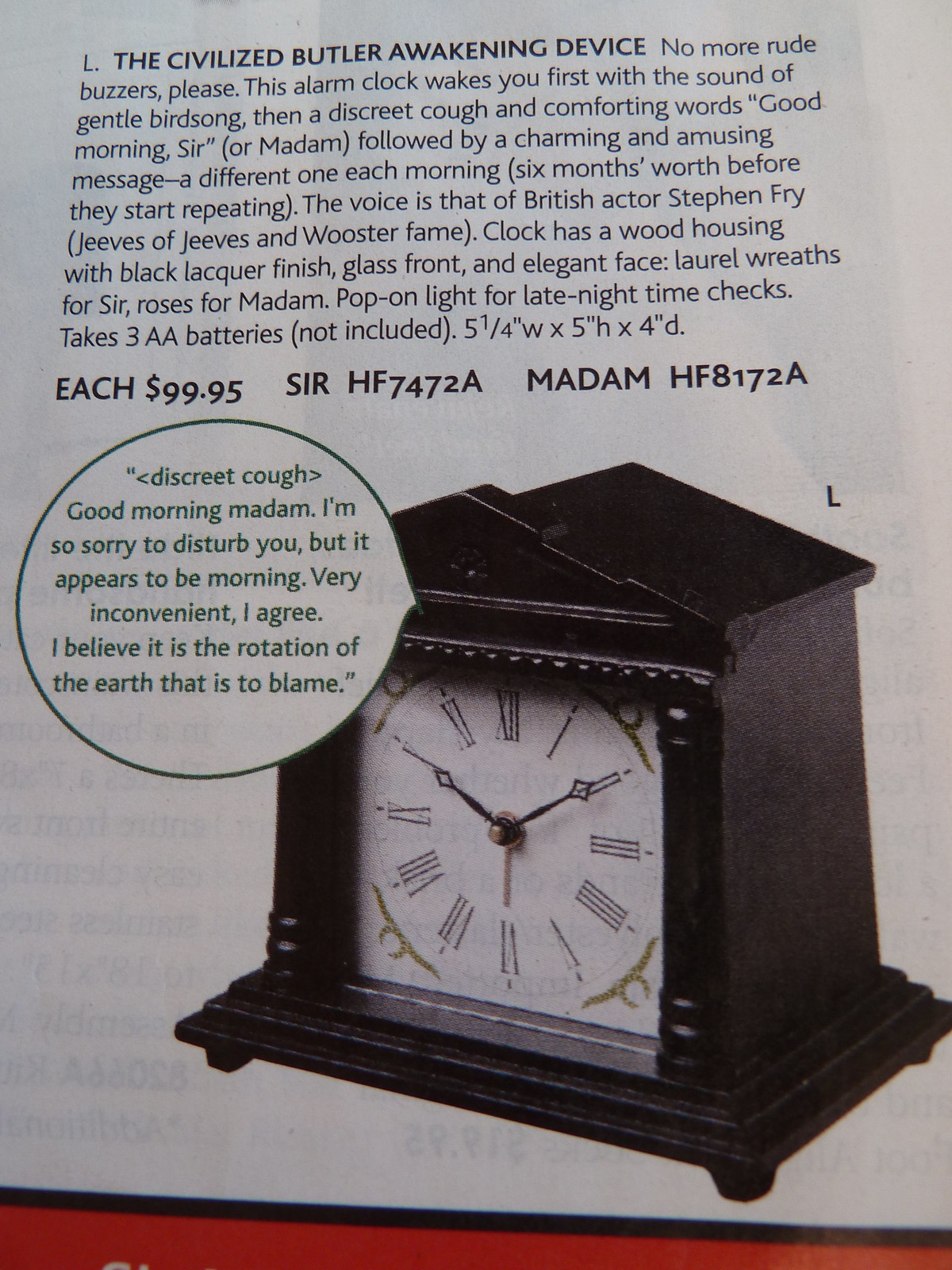This image is an advertisement for a distinctive alarm clock called "The Civilized Butler Awakening Device." The clock, resembling a small ornate desk clock with an old-style face and Roman numerals, is mounted on a pedestal and is designed to look like a miniature house. It features a wooden housing with a black lacquer finish, a glass front, and an elegant face adorned with laurel wreaths for "sir" and roses for "madam." 

At the top, the promotional text reads: "The Civilized Butler Awakening Device. No more rude buzzers, please." This sophisticated clock gently wakes the user with the sound of birdsong, followed by a discreet cough and then comforting words, "Good morning, sir or madam," delivered in the voice of British actor Stephen Fry, famous for role as Jeeves in "Jeeves and Wooster." The clock further charms with a different amusing message each morning, with a six-month cycle before repeating.

A speech bubble in the image humorously depicts the clock saying, "Good morning, madam. I'm sorry to disturb you, but it appears to be morning. Very inconvenient, I agree. I believe it is the rotation of the earth that is to blame." For nighttime convenience, the clock includes a pop-on light. 

The clock measures 5.25 inches in width, 5 inches in height, and 4 inches in depth. It requires three AA batteries, which are not included. Priced at $99.95 each, this alarm clock promises an elegant and gentle start to your day without the jarring sound of traditional buzzers.